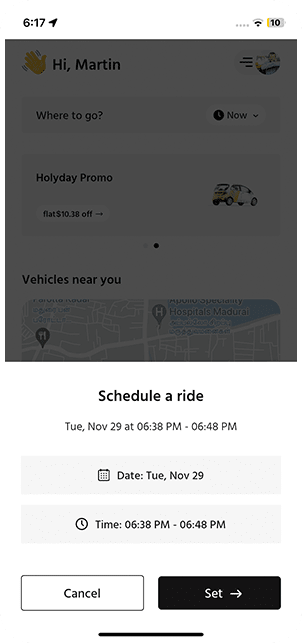**Detailed Caption:**

This is a vertically-oriented rectangular image, likely a screenshot taken from a smartphone. At the top left of the screen, "6:17" is displayed, accompanied by an arrow pointing slightly to the right. Moving towards the top right corner, there are four dots representing the network connection status, followed by a Wi-Fi signal icon showing three bars. To the right of the Wi-Fi icon, there are the numbers "3" and "10," likely indicating the current battery percentage and another status indicator.

Below the status bar, there is a large greyed-out box that occupies more than half of the image. Inside this box, the text "Hi Martin" is visible. To the left of the text, there is a clapping hands emoji, and to the right, a circular icon with a small image inside it. Further down within the greyed-out box, the text reads "Where to go" followed by "now," "holiday," and "promo." There is also a car icon next to the phrase "vehicles near you." Two small maps are also visible within this section, possibly indicating nearby locations or routes.

Beneath the large greyed-out box, there is a white background with the text "Schedule a ride Tuesday November 29th at 6:38 p.m. - 6:48 p.m." Below this, there is another grey box with "Tuesday November 29th" prominently displayed. Separated by a white line, there's another greyed-out section indicating a time range: "6:30 p.m. - 6:48 p.m."

The image provides a clear snapshot of scheduling details for a ride, complete with various interface elements indicating time, date, and possible promotional options.